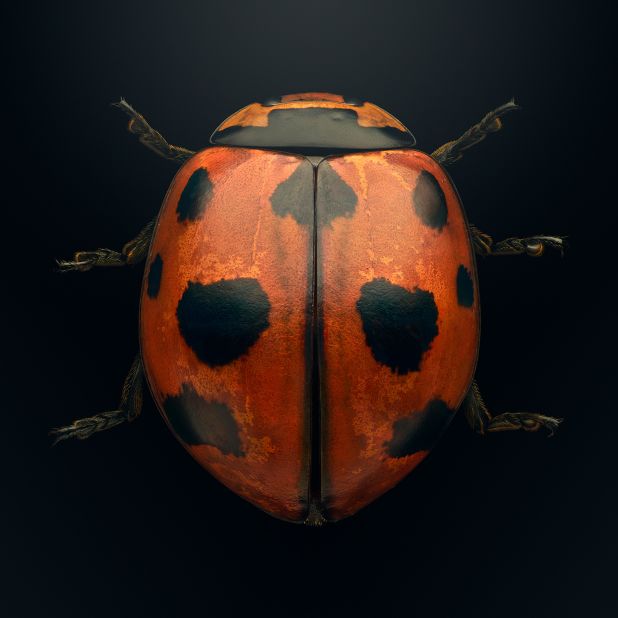This image focuses on an enlarged, highly detailed representation of a ladybug, also commonly known as a Japanese beetle or lady beetle. The ladybug is viewed from a top-down perspective against a pitch-black background, emphasizing its vibrant coloration. The head is positioned towards the top of the frame, with the tail towards the bottom. The insect's body is predominantly a dark orange to yellowish-orange shade, accented with several black spots of varying shapes, creating an almost symmetrical pattern on either side. The ladybug features six legs, visibly extending outward, and a distinct line that runs down the middle of its elytra, indicating where the wings would separate. Its eyes are clearly visible near the top center of the image, near a lighter orange region of the head, which also includes a black collar-like marking. The meticulous details, from the splotchy dots to the light and dark orange hues and specific anatomical features, give the impression of a piece of art rather than a mere photograph.